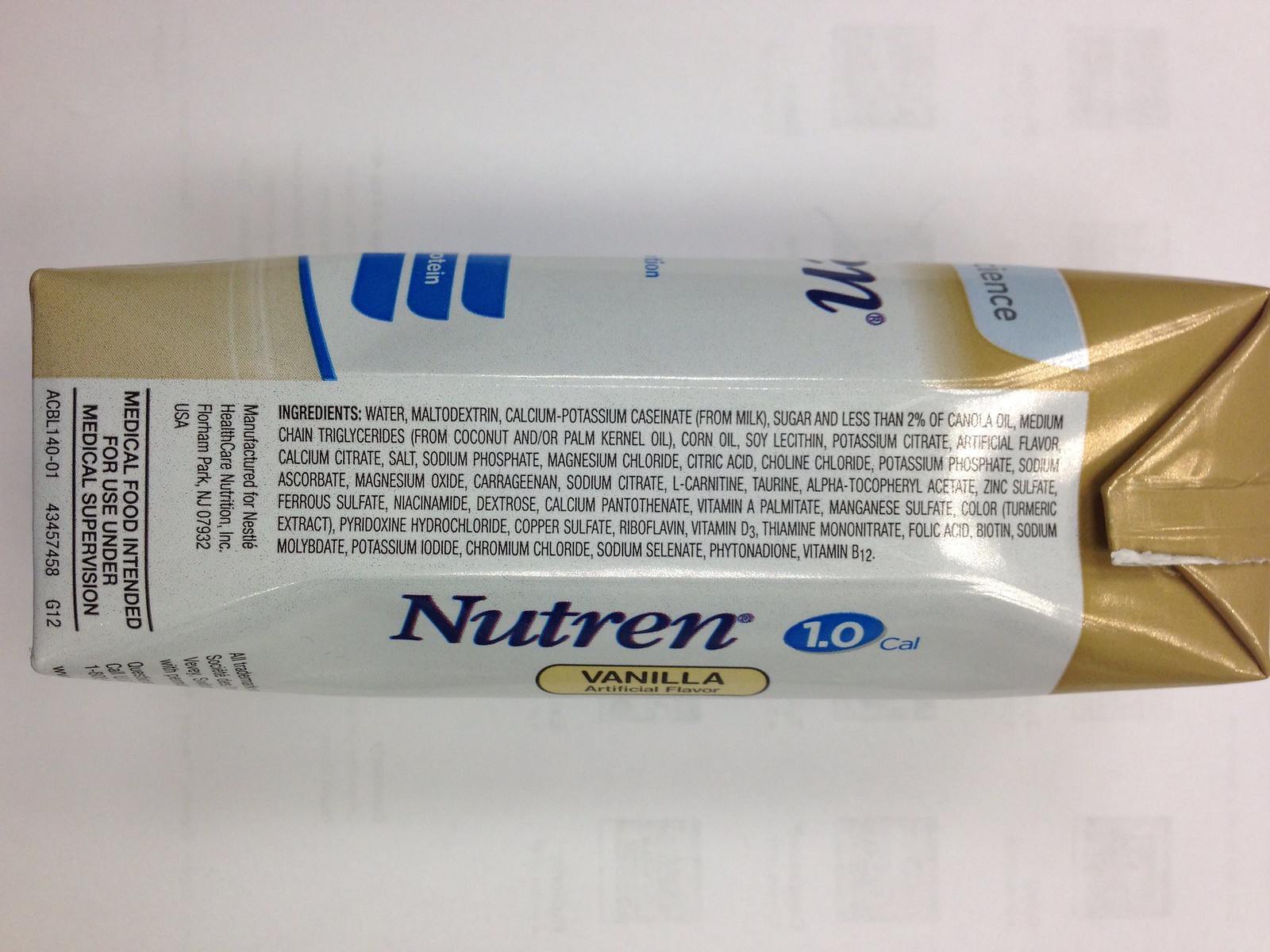The image depicts a nutrition drink package laying on its side atop a white surface, displaying the nutrition facts and ingredients prominently. The package features a gold, white, and blue color scheme with blue and black text. The product name "Nutrin" is printed in navy blue, followed by "1.0 CAL" with "1.0" inside a blue circle and "CAL" in smaller blue letters. The flavor, indicated as vanilla with artificial flavoring, is written in black against a tan-colored background. This medical food, intended for use under medical supervision, is manufactured for Nestle Healthcare Nutrition in New Jersey. The package appears heavily laminated with plastic, giving it a glossy look. The background reveals faint, sketch-like illustrations visible through the white surface.